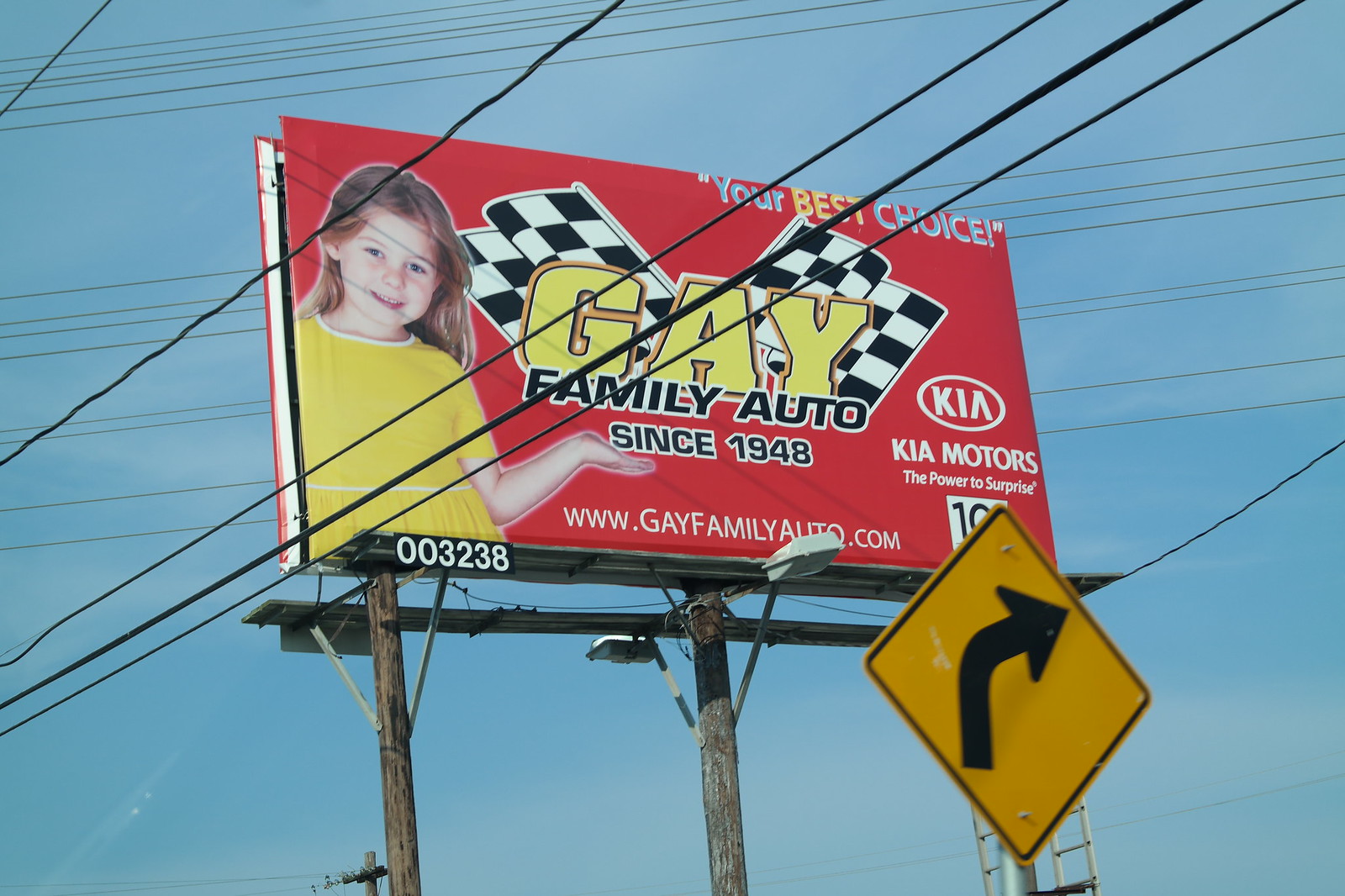The billboard prominently features the text "Gay Family Auto Since 1948," with the word "Gay" displayed in large, bold yellow letters. The phrase "Family Auto Since 1948" is written in smaller black text. Behind the word "Gay," two checkered flags are crossed, adding a dynamic element to the design. The slogan "Your Best Choice" appears on the billboard, with "Your" and "Choice" in blue letters and "Best" in yellow.

On the left side of the billboard, there is an image of a young girl making a hand gesture as if she is serving, contributing a welcoming and friendly touch. At the bottom of the billboard, the website "www.gayfamilyauto.com" is printed in white text, encouraging viewers to visit the site for more information. In the upper right corner, the Kia Motors logo and the tagline "The Power to Surprise" are displayed.

The background of the billboard is a striking red, enhancing the overall visibility and emphasizing the key messages. Surrounding the billboard are numerous power lines, indicating a busy or urban setting. In the foreground, at the bottom of the scene, there is a yellow "Veer to the Right" traffic sign with a black arrow, directing drivers on the adjacent road.